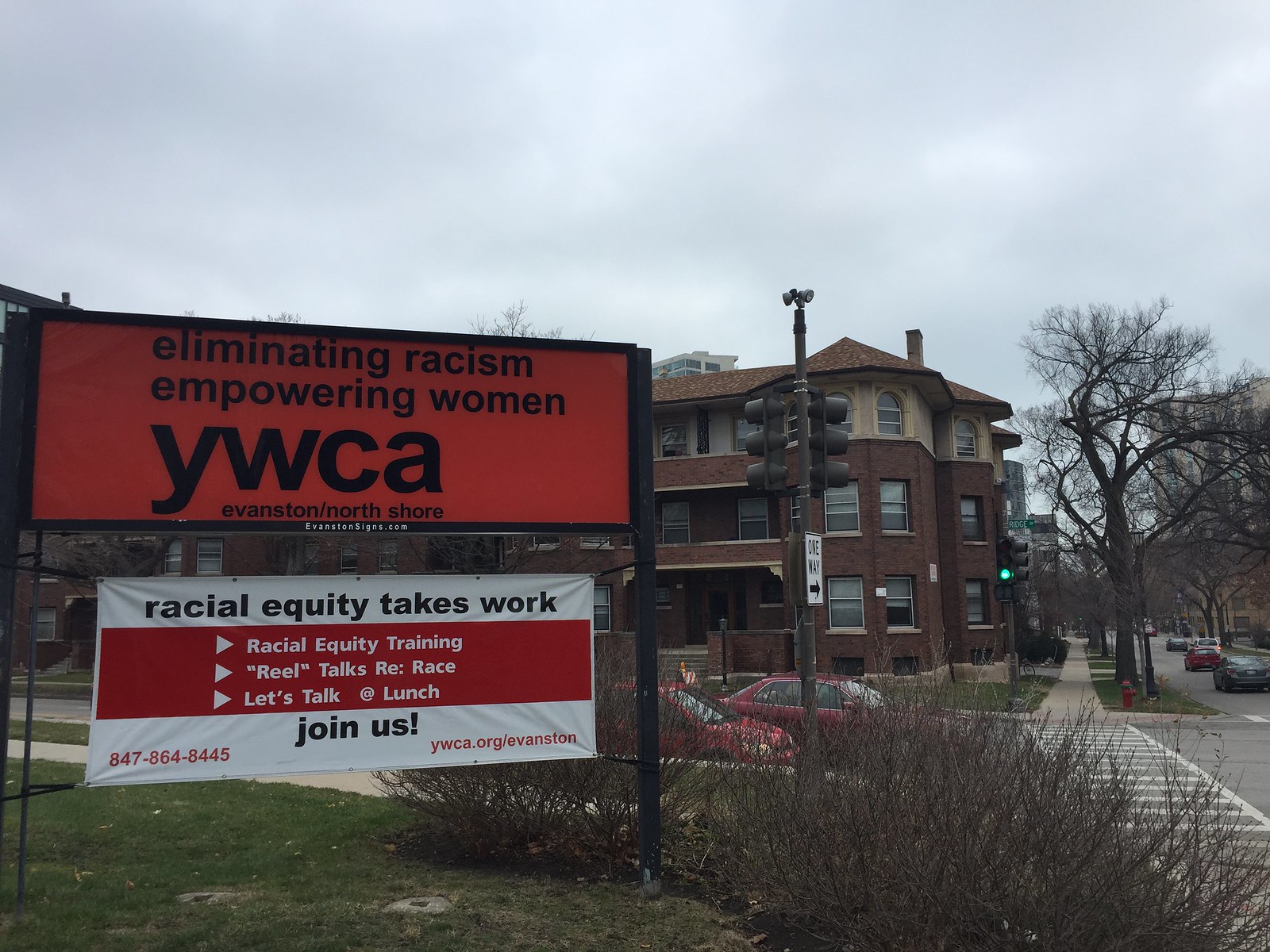The image depicts a street scene with a prominent red and white sign from the YWCA Evanston/North Shore. The top of the sign displays the messages "Eliminating Racism" and "Empowering Women," followed by "YWCA" on a reddish background. Beneath that, a banner reads "Racial Equity Takes Work" with additional information including "Racial Equity Training," "Real Talks on Race," and "Let's Talk at Lunch," all encouraging community involvement with the phrase "Join Us!" and a contact phone number. The sign also features the URL: YWCA.org/Evanston.

The setting appears to be in late fall or early winter, with trees stripped of leaves lining the street. A shrub and grass are visible at the forefront of the image. In the background, there is a light gray sky and a Tudor-style building that may be apartments. Cars are seen driving down the street and at a nearby crosswalk. A one-way street sign is present, adding to the urban environment.